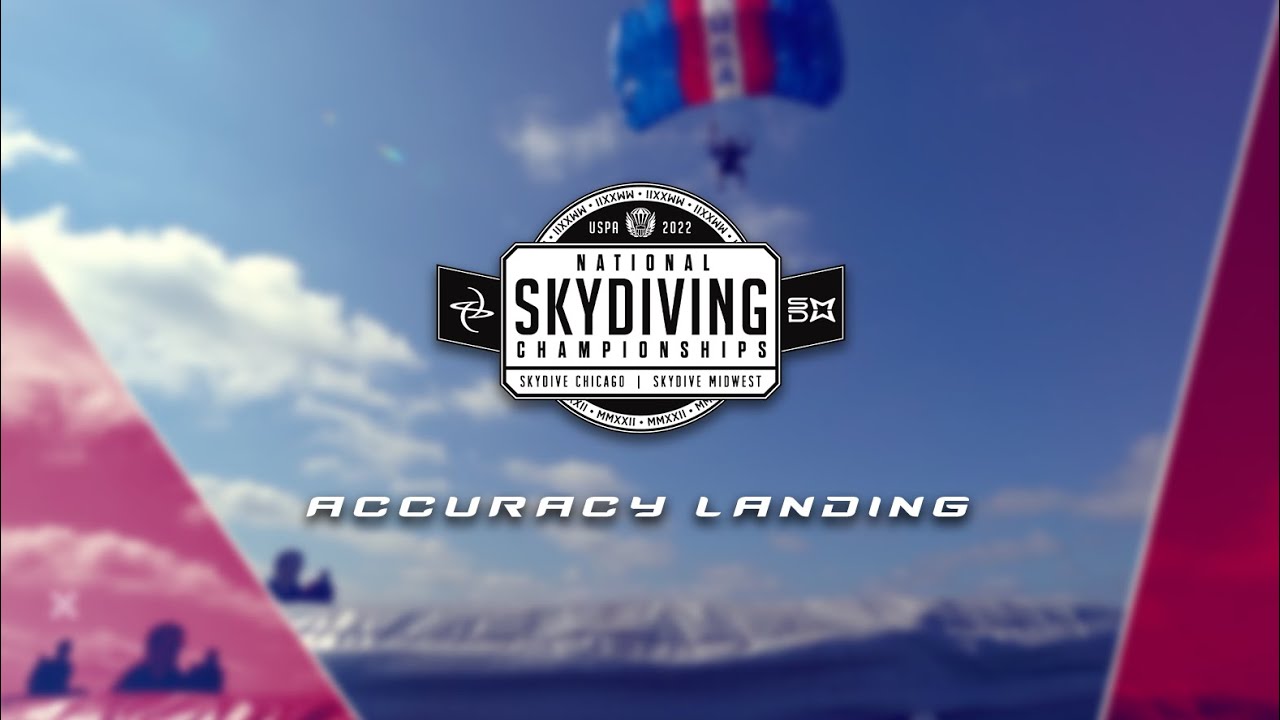The image is a detailed promotional piece for the National Skydiving Championships, likely a screenshot from a video. Central to the composition is a bold rectangular logo with chunky beveled edges, resembling a license plate font, that reads: "National Skydiving Championships, Skydive Chicago, Skydive Midwest." Positioned at the top of this logo is "USPA 2022," signifying the event year, and it sits within a circular emblem featuring additional details in Roman numerals along the rim.

Below the main logo, the text "Accuracy Landing" stands out in a futuristic Blade Runner-esque font. The visual is accentuated with a striking image of a skydiver descending with a blue and red parachute featuring a white color block that appears to spell out "USA." This action scene unfolds against a backdrop of snow-capped mountains and a clear blue sky, dotted with clouds on the left, reinforcing the dramatic and picturesque setting. The overall design, with its intricate logos and dynamic imagery, encapsulates the thrilling essence of the National Skydiving Championships.